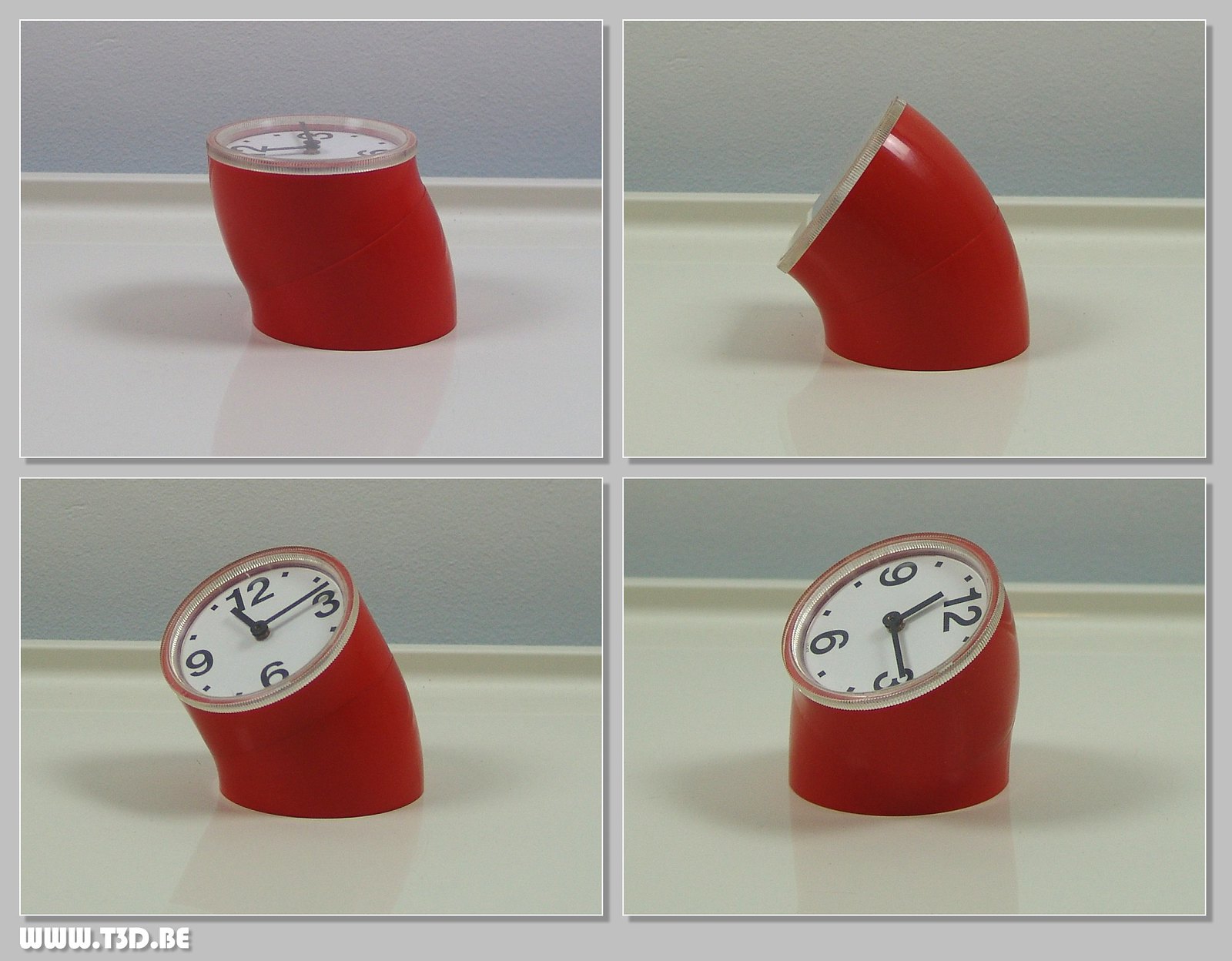The image showcases a unique clock presented in a grid of four separate squares, each displaying the clock from different angles. The clock is mounted on a peculiar, thick red base resembling a flexible, twisted tube, similar to a slinky or serpentine shape. This red base, made of plastic or rubber, features an adjustable design, allowing the clock's position to be altered and twisted into various configurations. The clock face, which is at the top of the red base, is white and prominently displays the numbers 12, 3, 6, and 9 in black. It includes both an hour hand and a minute hand, protected under clear plastic for visibility. The four images in the grid highlight different perspectives of the clock: the top left image shows more of the red base with a hint of the clock face, the top right image emphasizes the curved nature of the red base with the clock encased in plastic, and the bottom images illustrate the clock in slightly slanted positions, showcasing the base's adaptability. A small text in the bottom left corner reads www.t3d.be, suggesting a possible source or branding.